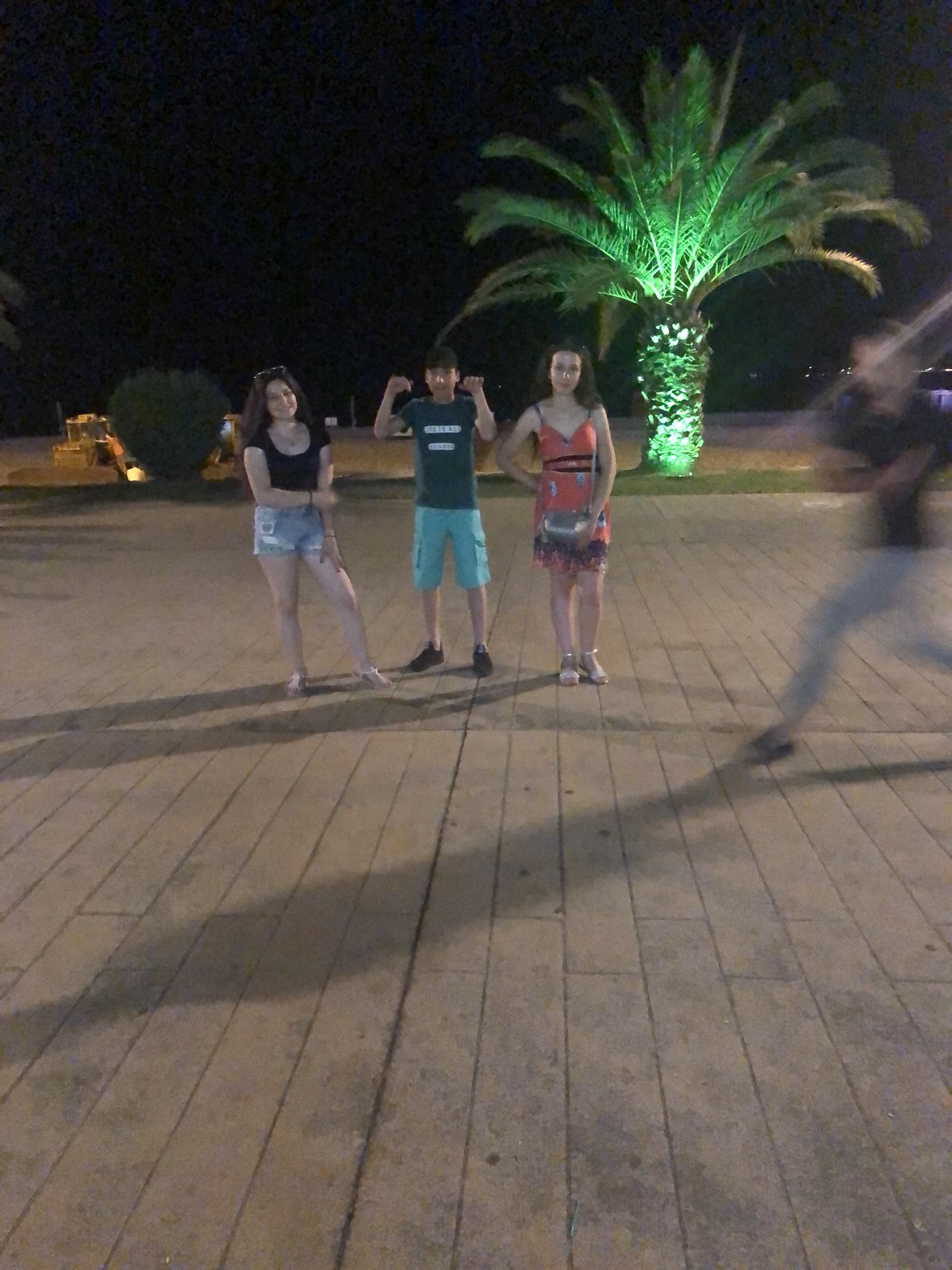This photograph captures a lively moment on a wooden walkway at night. In the center of the image, three teenagers are posing as if for a portrait. On the left stands a young girl with long brown hair, a black shirt, short jean shorts, and white sandals. She also has glasses resting on top of her head. Beside her in the middle is a boy wearing a green shirt with writing on it, light blue cargo shorts, and black tennis shoes; he has dark hair or possibly a hat on, and his arms are raised in a playful gesture. On his right is another girl with brown hair, dressed in a vibrant red dress with black accents and a black belt, also wearing white sandals. She carries a cross-body purse, with one hand behind her back. Adding to the dynamic scene, on the far right, another person seems to be hastily running through the shot, appearing as a blur in gray pants and a black shirt. The background features an illuminated palm tree with greenish lights, a dark green bush on the left, and the night sky, creating a vibrant and energetic atmosphere.